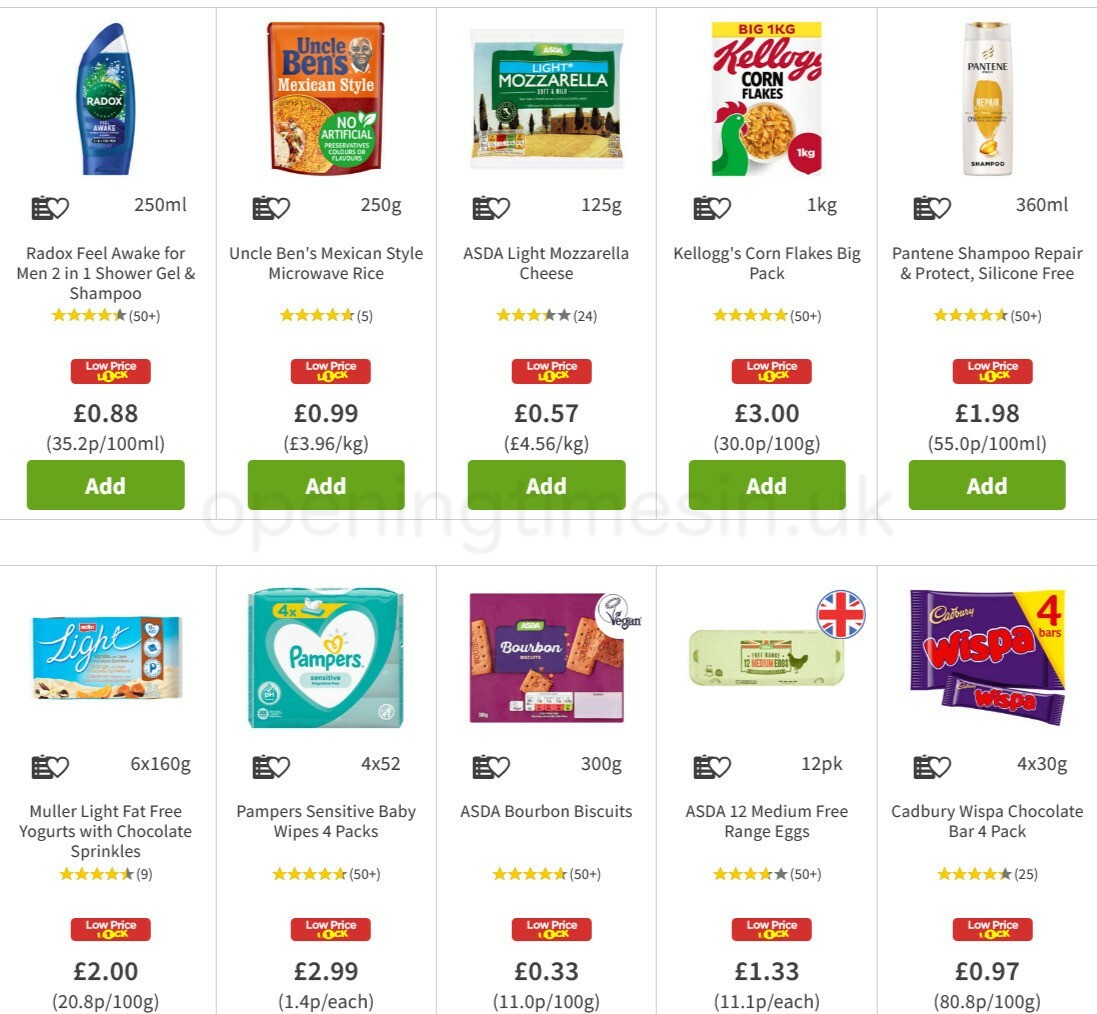This image appears to be a screenshot from an online shopping website displaying various products in a grid layout. The grid consists of 5 columns and 2 rows of items. Here is a detailed breakdown of the items listed:

**Top Row (Left to Right):**
1. **Radox Feel Awake for Men 2-in-1 Gel and Shampoo**
   - Rating: Visible
   - Price: £0.88
   - Add to Cart Button: Green

2. **Uncle Ben's Mexican Style Rice**
   - Rating: Not specified
   - Price: Visible
   - Add to Cart Button: Green

3. **ASDA Light Mozzarella Cheese**
   - Product: Light Mozzarella
   - Rating: Visible
   - Price: Not specified
   - Add to Cart Button: Green

4. **Kellogg's Corn Flakes (1kg)**
   - Rating: Not specified
   - Price: £3.00
   - Add to Cart Button: Green

5. **Pantene Shampoo Repair and Protect Silicone Free**
   - Rating: Visible
   - Price: £1.98
   - Add to Cart Button: Green

**Bottom Row (Left to Right):**
1. **Mueller's Light Fat-Free Yogurts with Chocolate Sprinkles**
   - Rating: Visible
   - Price: £2.00
   - Add to Cart Button: Partially cut off

2. **Pamper's Sensitive Baby Wipes 4-pack**
   - Rating: Not specified
   - Price: £2.99
   - Add to Cart Button: Green

3. **ASDA Bourbon Biscuits**
   - Rating: Not specified
   - Price: £0.33
   - Add to Cart Button: Green

4. **ASDA 12 Medium Free Range Eggs**
   - Rating: Visible
   - Price: £1.33
   - Add to Cart Button: Green

5. **Cadbury Wispa Chocolate Bar 4-pack**
   - Rating: Visible
   - Price: £0.97
   - Add to Cart Button: Green

Each item is displayed with a visible rating and an 'Add to Cart' button, facilitating easy shopping.